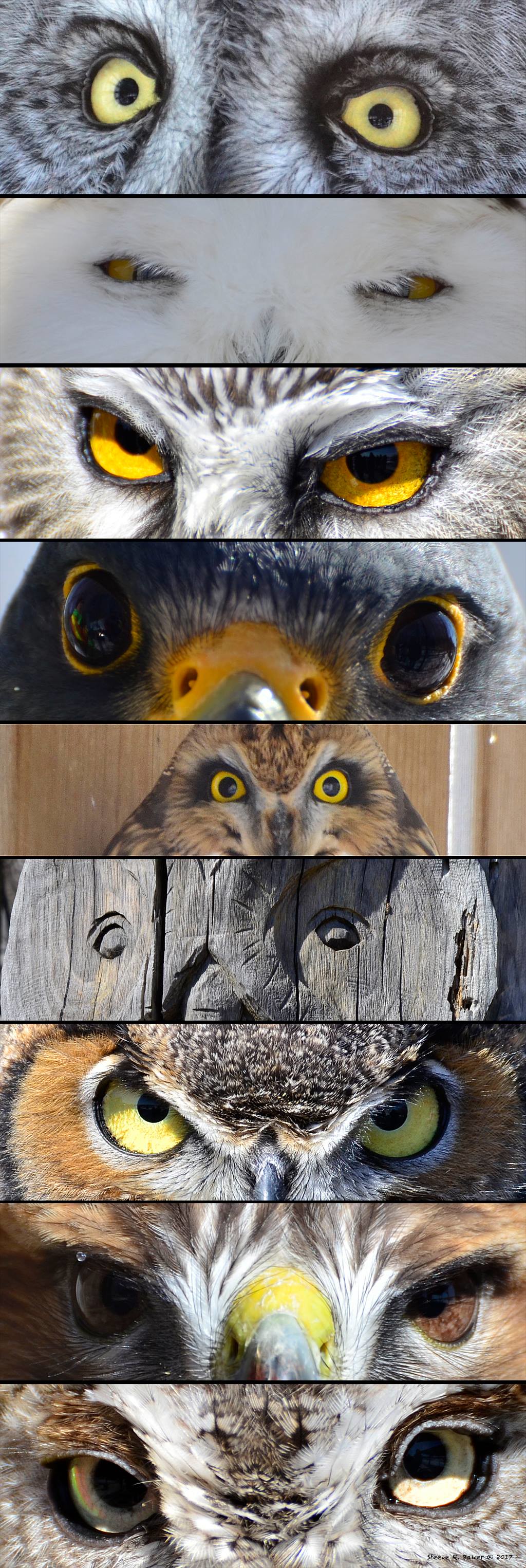This detailed composite image presents a vertical collage of various birds of prey's eyes, creating an intense and captivating visual akin to a totem pole. Starting from the top, the first close-up shows the piercing yellow eyes of an owl with a greyish hue. Directly below, a snowy owl with squinted yellow eyes and white feathers is prominently featured. The third close-up is a more typical brown owl, distinguished by its sharp yellow eyes and characteristic features. Following this owl, the image includes the fierce gaze of a hawk or an eagle, noticeable by its black eyes and yellow beak.

In the middle of the collage, a shift occurs with a strikingly weathered piece of wood, featuring two knots resembling eyes, evoking a sense of a carved owl. Below this wooden anomaly, the pattern continues with another close-up of an owl, where the yellow eyes once more dominate. A bit further down, the eyes of a brown and white hawk, with greenish undertones, stare out with predatory intensity. The sequence finalizes with an owl showcasing whitish-yellow eyes, merging the collage into a cohesive yet diverse representation of avian predators.